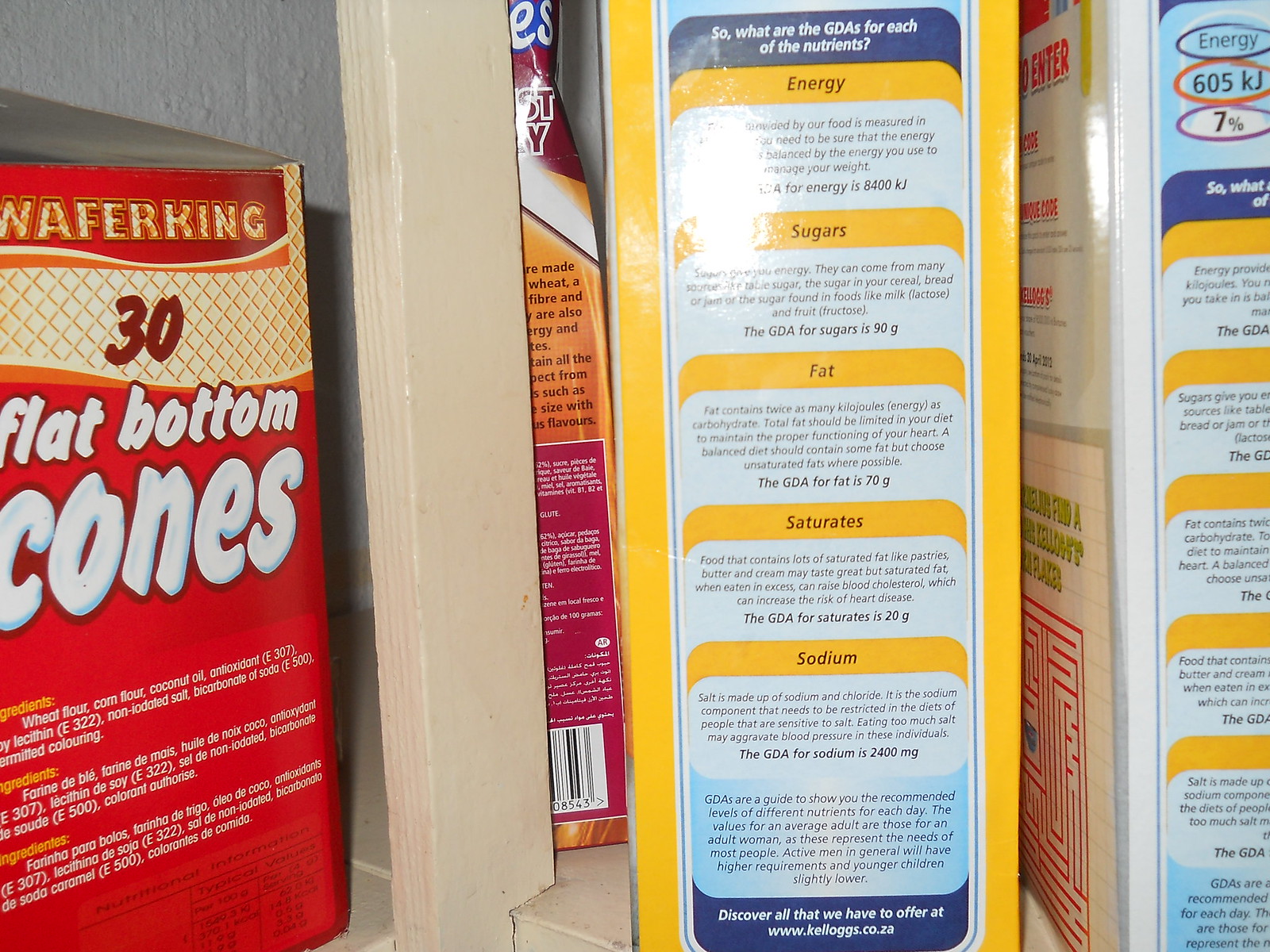The image captures a neatly arranged pantry shelf filled with an assortment of food boxes. On the left-hand side, prominently featured is a vibrant red box adorned with orange, yellow, and white lettering that reads "Flat Bottom Cones." This box, labeled "Wafer King" and containing 30 cones, goes further to list its ingredients. Nestled amidst the other boxes, a slightly crushed red and orange box can be seen in the corner, though only partial text is visible showing "ES" and "STY." In front of this, another box is positioned spine-out, displaying the text, "So what are the GDAs for each of the nutrients?" It details energy, sugars, fat, saturates, and sodium, each with a brief paragraph. Further to the right, a white box with light blue lettering indicates "Energy 605 KJ, 7%," and features a small red maze on its back panel. This organized yet eclectic mix of boxes provides a glimpse into a well-stocked pantry.